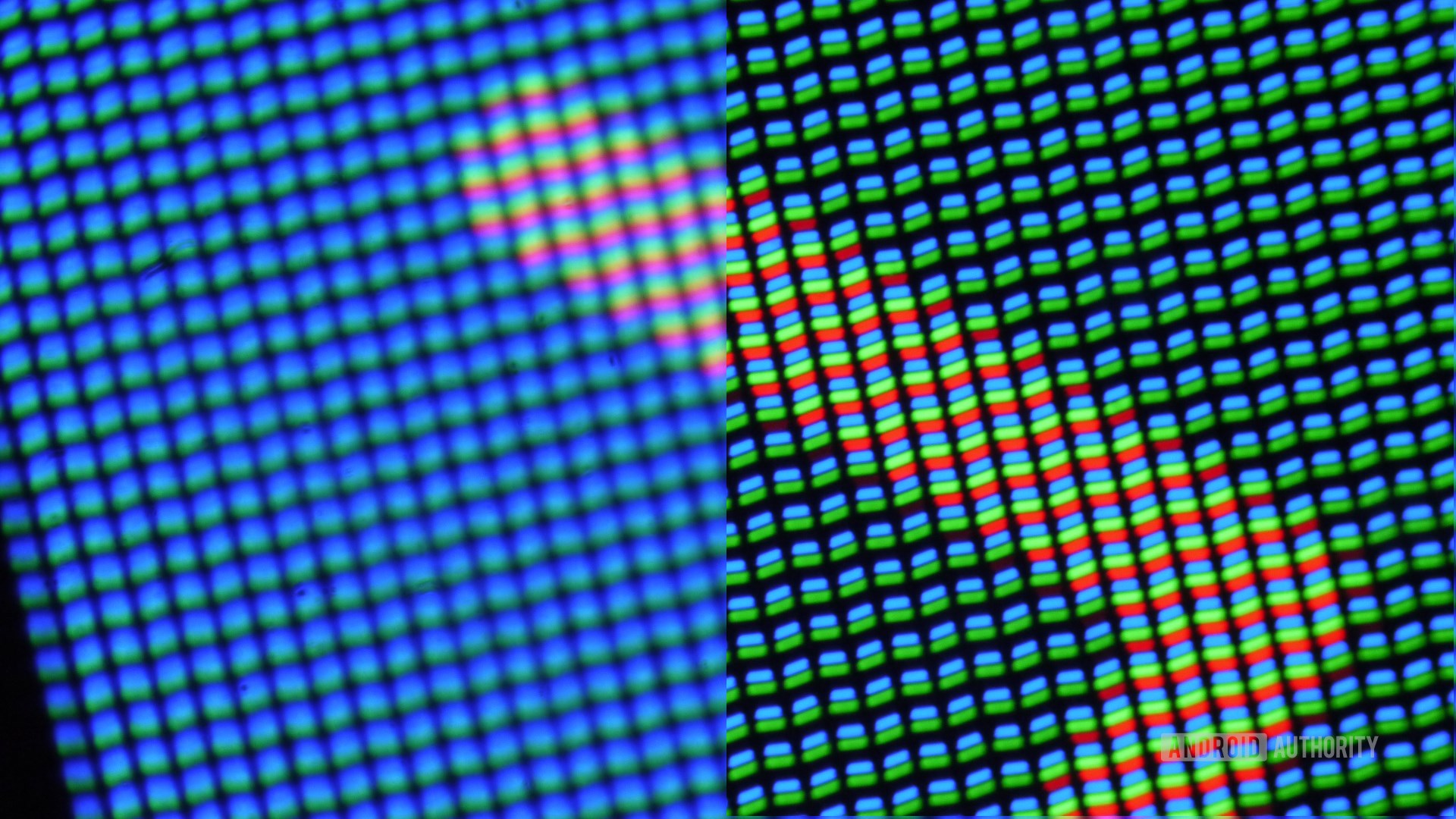This close-up photograph captures a pixelated screen displaying an intricate mosaic pattern comprised of small squares. On the left side, the image is slightly blurred, showcasing an askew arrangement of blue and green squares, with each square featuring a green bottom and a blue top, set against a completely black backdrop. The right side of the image is sharply in focus, featuring a similar pattern punctuated by a vibrant, rotated L-shaped figure that appears to the left, with significantly brighter blue and green colors alongside red rectangles between the squares. Additionally, there’s a faint watermark on the bottom right corner that reads "Android Authority" in white. The word 'Android' is inverted, outlined by a white rectangle with the text cut out, while 'Authority' is written in standard white text. The mosaic is rendered with intricate black lines separating each square, and a noticeable yellowish tan line runs diagonally across the top, transitioning smoothly from the blue section to the green section, culminating in the bottom right corner.